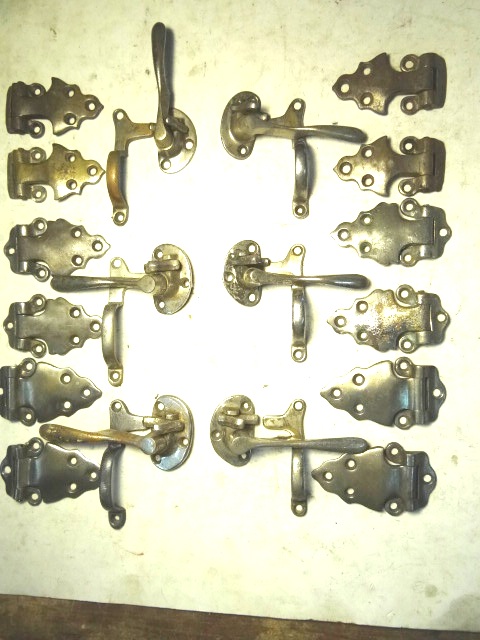This photograph captures an array of antique brass hardware meticulously arranged against an off-white surface. The collection includes over a dozen pieces, featuring various types of latches, hinges, and doorknobs that exude an old-fashioned charm. The hardware appears aged, with a patina and slight discoloration giving each piece a unique, timeworn character. Among the items are approximately ten decorative hinges with a distinct wavy design, and possibly door handles, arranged in orderly columns. Some hinges consist of two parts, one resembling a lever and the other a small handle. The setting is indoors, and the overall composition is rectangular, showcasing the intricate details and vintage allure of these brass fixtures.